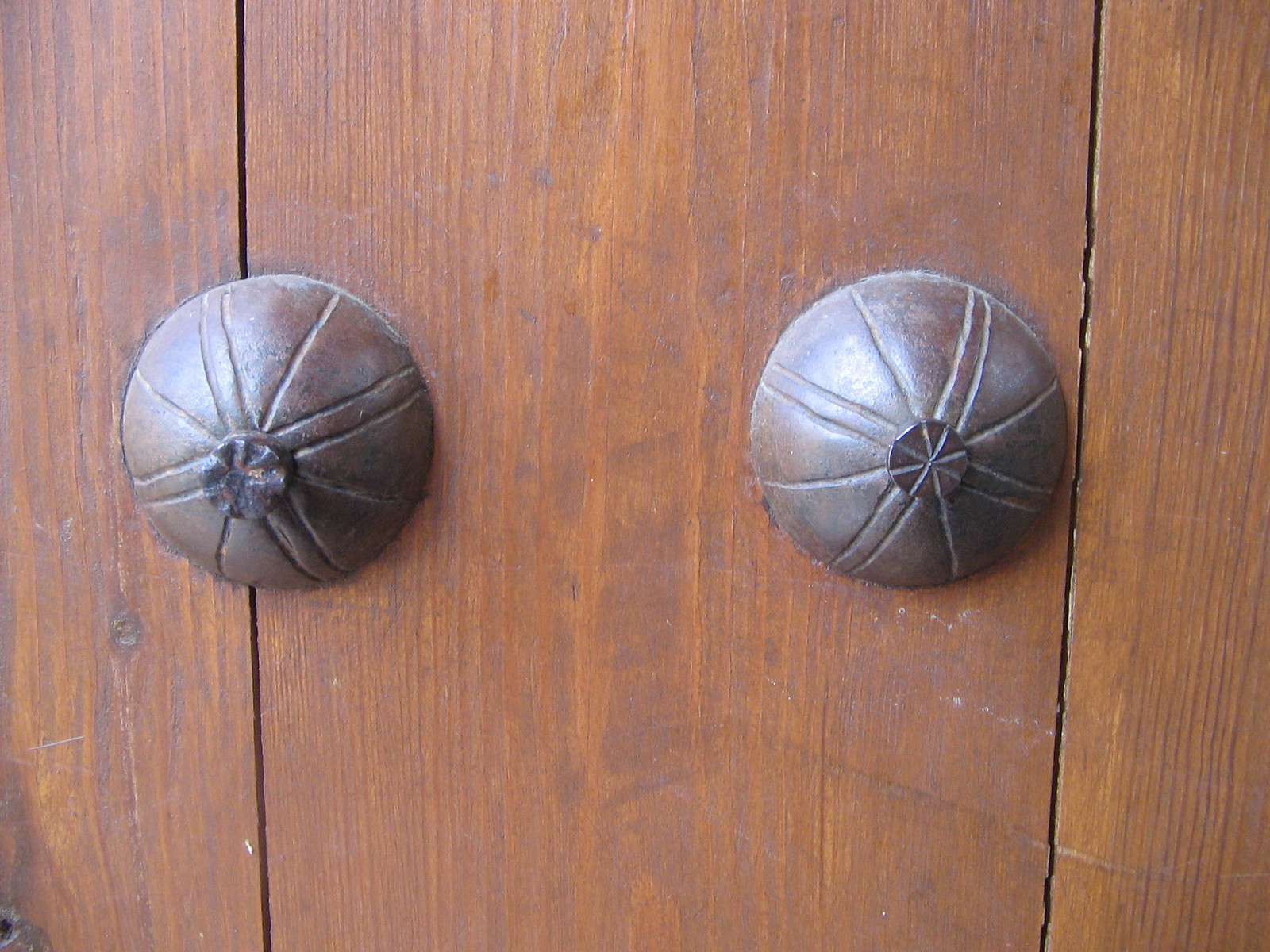This photograph features a pair of dark brown, possibly oak, wooden planks with two attached half-sphere shapes that look like bronze-colored metal. These shapes, about four inches in diameter, contain intricate designs: they have lines forming a pattern that includes both double lines and a plus sign or X shape. Each half-sphere has a knob at its center, also detailed with lines, though the one on the left appears more worn than its counterpart. These elements suggest the structure might function as a cabinet door, though no hinges are visible.